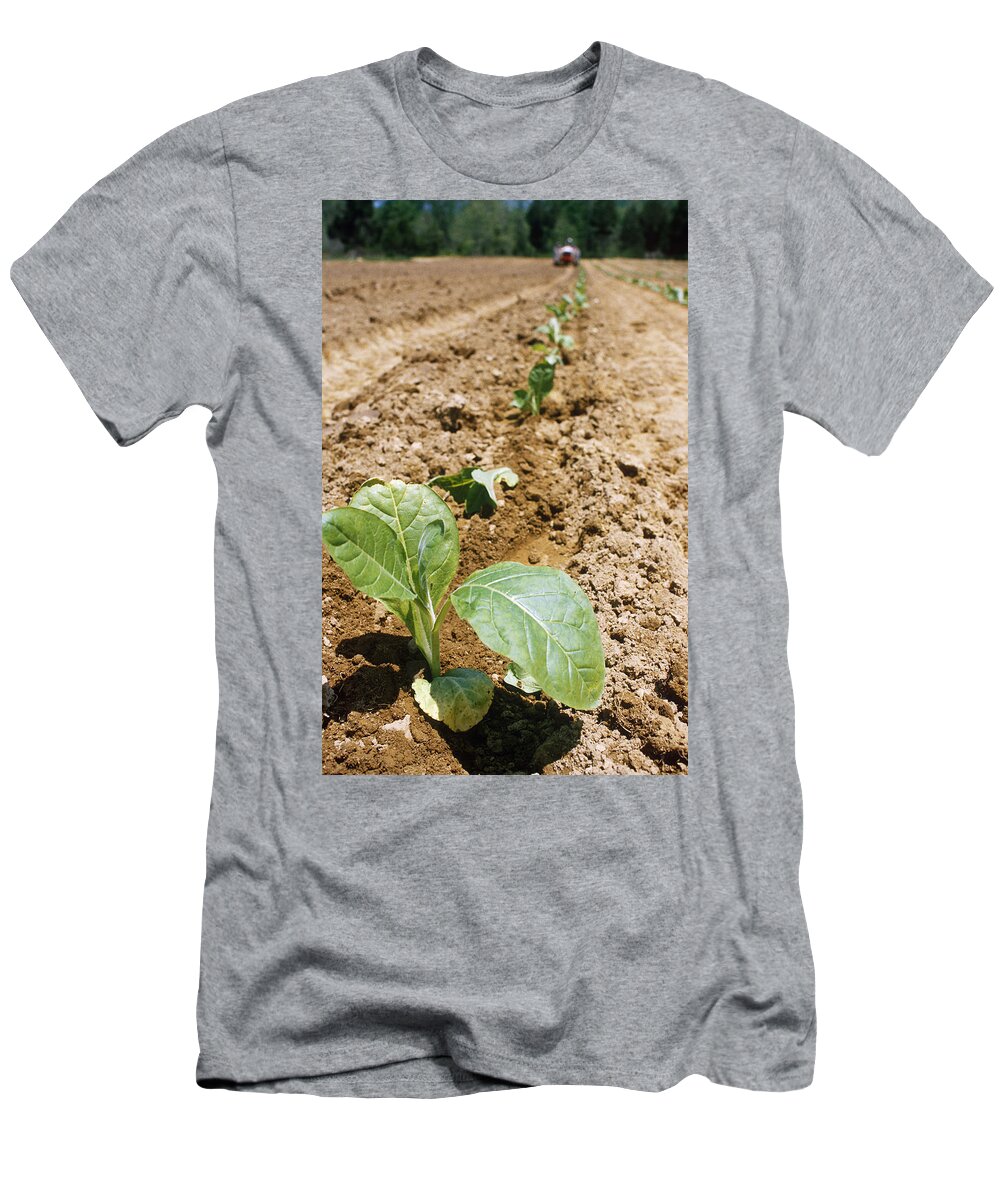This image showcases a short-sleeved, crewneck gray t-shirt, laid on a white background. The shirt itself is somewhat wrinkled and rumpled, not lying completely flat. A rectangular, vertically-oriented image is printed on the front of the shirt, just below the collar, and appears slightly awkwardly placed.

The image on the t-shirt is a detailed photograph of a plant growing from the soil. The shot is taken in portrait mode, focusing on the young green sprouts emerging from the ground. The soil is dark brown where the seeds have been planted, surrounded by lighter brown dirt. In the blurred background, farm soil, possibly on a field, stretches out with various green plants populating the space, showing clear signs of agricultural activity. Additionally, a small, somewhat indistinct tractor can be seen in the distance, accompanied by a range of trees in different shades of green, from light to dark. The attention to detail captures not only the emerging sprouts but also the environment around them, suggesting a scene from a farm with ongoing cultivation.